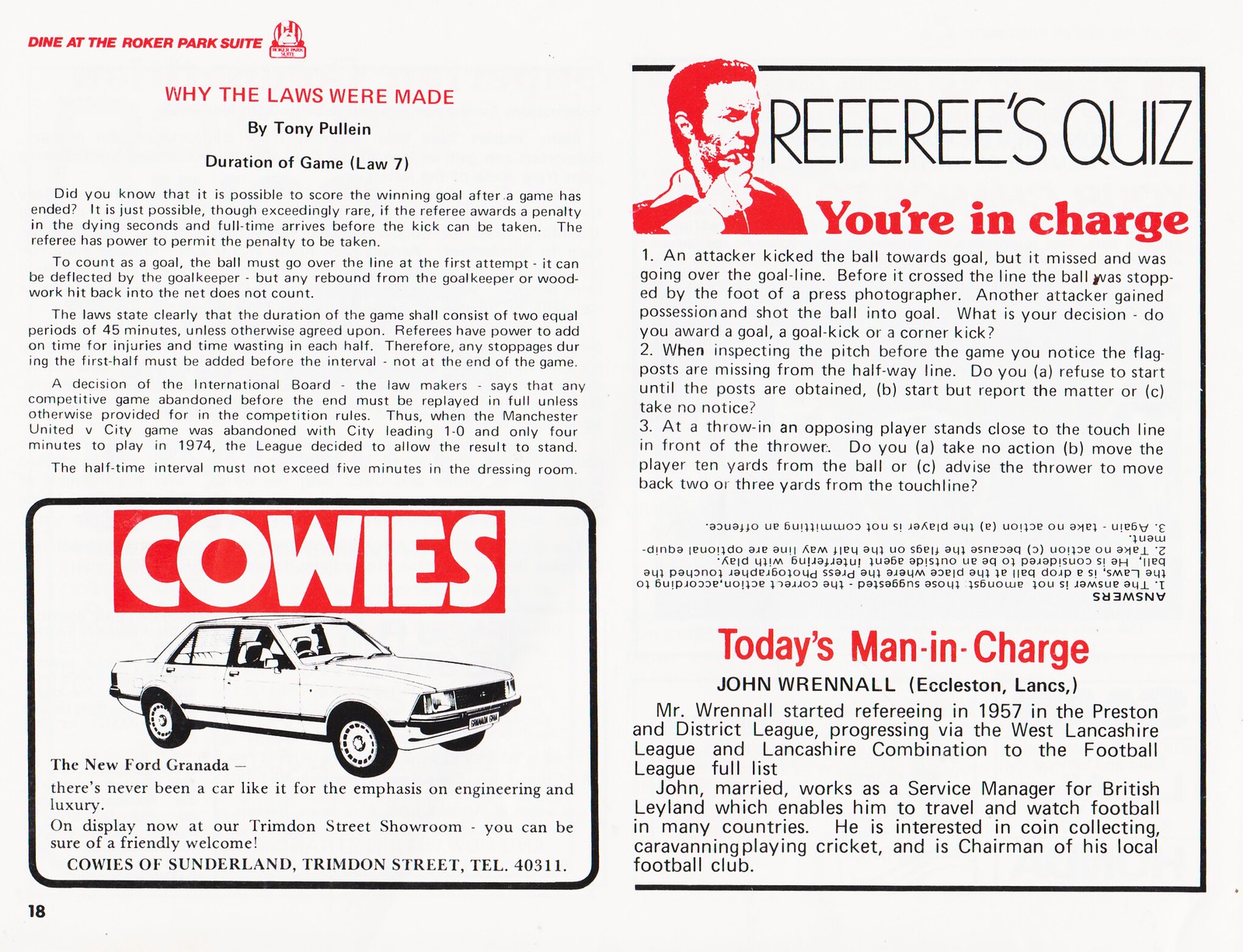The image shows the inside pages of an old magazine or brochure filled with several articles and advertisements. Dominating the top left corner is a banner reading "Dine at the Roker Park Suite," accompanied by what appears to be an illustration or icon of the building. Below that, an article titled "Why the Laws Were Made by Tony Pullian, Duration of Game, Law 7" begins with the intriguing fact, "Did you know that it's possible to score the winning goal after the game has ended?" Further text ensues, making for a dense read. Positioned prominently in the bottom left corner is an advertisement for "The New Ford Granada," courtesy of Cowies of Sunderland, featuring a white car angled left-to-right and accompanied by contact details in a red box with large white capital letters.

In the top right, the headline "Referee's Quiz, You're in Charge" is displayed with a black-and-white image of a man with a whistle in his mouth. The quiz poses a scenario: "An attacker kicked the ball towards the goal, but it missed and was going over the goal line. Before it crossed the line, the ball was stopped by the foot of a press photographer. Another attacker gained possession and shot the ball into the goal. What is your decision? Do you award the goal? A goal kick or a corner kick?" It further challenges readers with, "When inspecting the pitch before a game, you notice the flag posts are missing from the halfway line. Do you refuse to start until the posts are obtained, start but report the matter, or take no notice?" Below this section, there is an article titled "Today's Man in Charge" by John Ronald Reynolds from Eccleston, Lancs, featuring several paragraphs about him.

The colors in the image are a mix of black, white, and red, with hints of gray, giving it an old-school, textbook-like appearance.